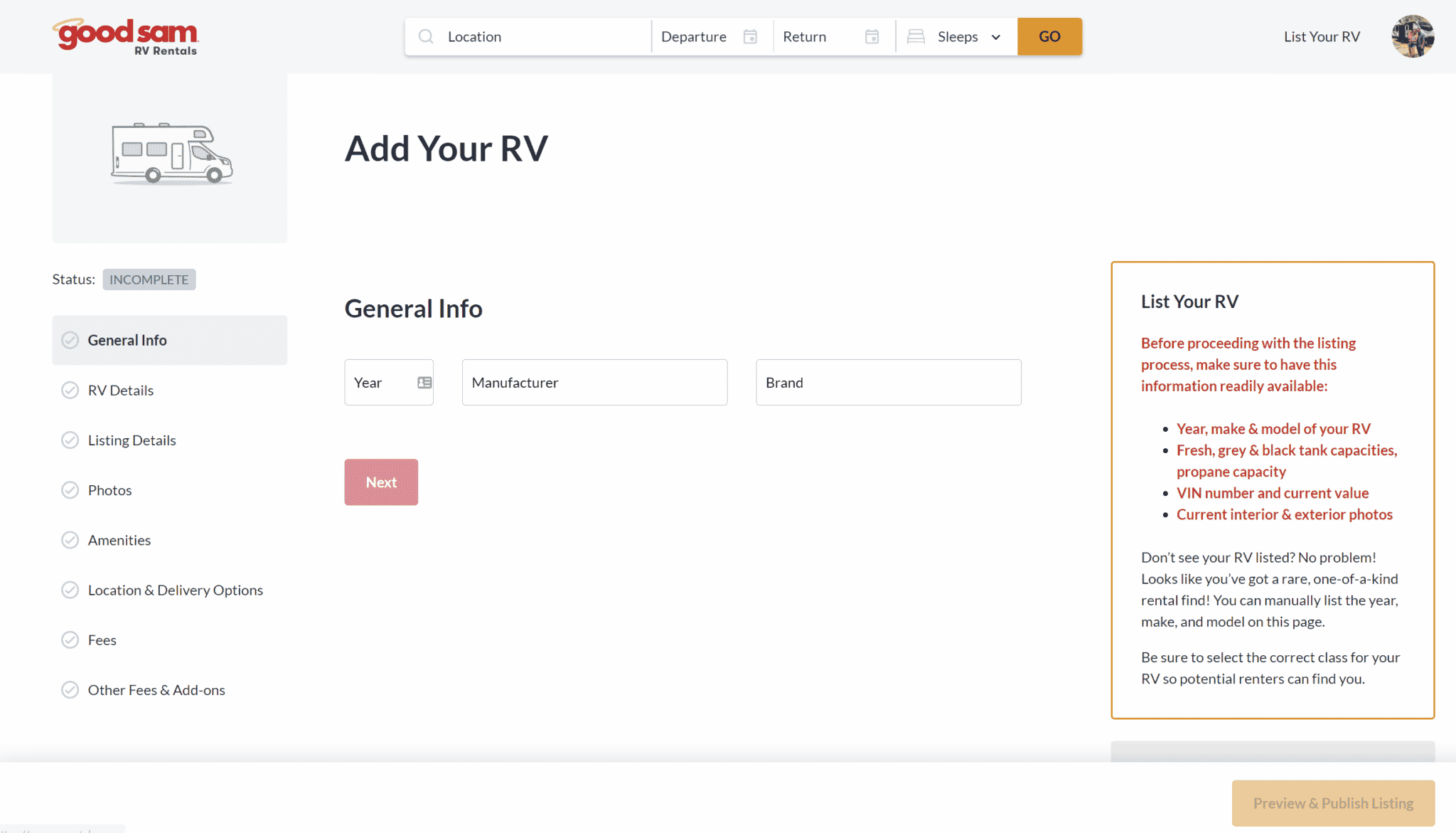A detailed webpage from Good Sam, a popular RV rental platform, is displayed. The top section prominently features navigation options, including fields for 'Location,' 'Departure,' 'Return,' and 'Sleeps,' which help users find and filter available RVs. On the right side, there's an option to 'List Your RV,' suggesting that users can rent out or sell their RVs through the site. Clicking this option reveals requirements for listing an RV, such as the year and make of the vehicle, fresh water tank capacities, propane levels, VIN number, and current value, along with interior and exterior photos.

A profile picture is visible, indicating the user is logged into their account. Below, the site outlines several steps and sections to complete the listing process: 'General Info,' 'RV Details,' 'Listing Details,' 'Photos,' 'Amenities,' 'Commission and Delivery Options,' 'Fees and Other Fees,' and 'Add-Ons.' This structured menu ensures that all necessary information is provided for potential renters to evaluate an RV. The comprehensive guidance and detailed fields make it clear and straightforward for users to list their RVs for rent.